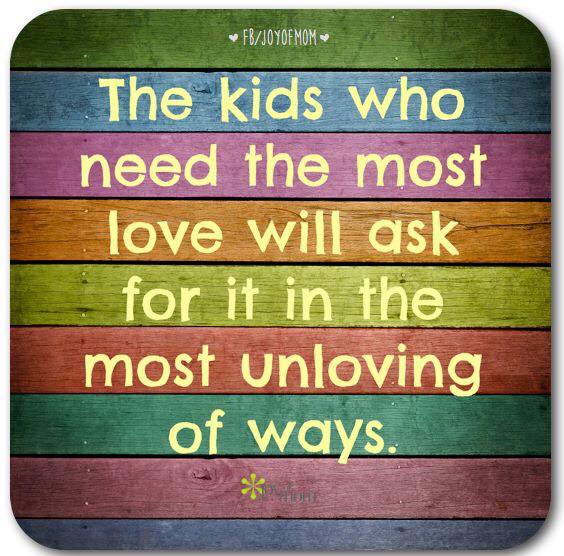This image is a heartwarming and colorful square graphic often shared on social media, attributed to "Joy of Mom." The central text reads, "The kids who need the most love will ask for it in the most unloving of ways," written in clean white font. Above the text, there's a heart icon followed by the link "FB/joy of mom," also in white. The background consists of horizontal wooden planks or blocks, stacked in vibrant, varied colors: dark green, light blue, light purple, dark yellow, light green, dark pink, dark green, dark pink, and dark blue, creating a rich rainbow effect. The image has a charming appearance with rounded corners, adding to its approachable and sweet design.